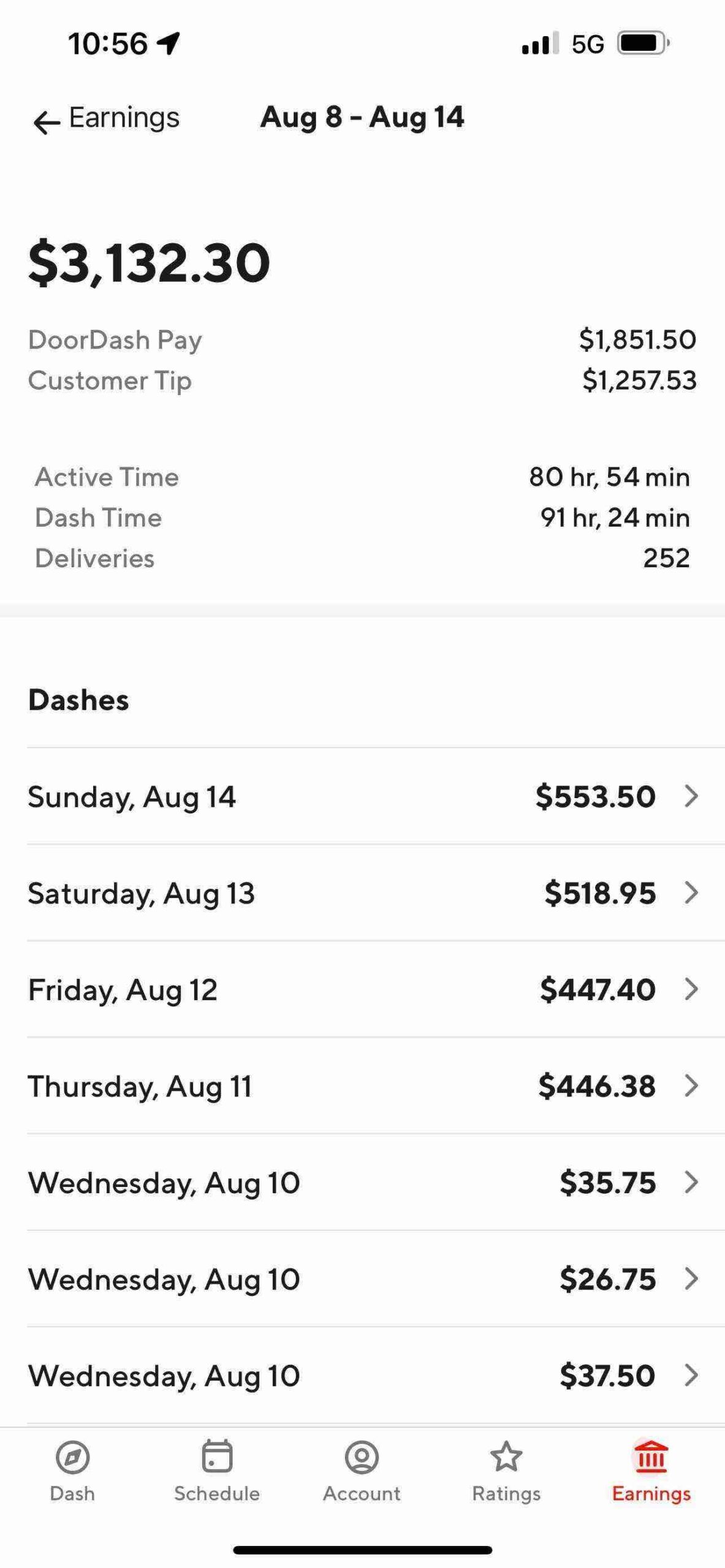The image displays a detailed payment summary for an individual working as a DoorDash delivery driver, visible on a cell phone screen. At the top of the screen, the cell phone status bar shows the battery meter, clock, and signal strength indicators. Directly below this bar, the title "Earnings" is displayed, followed by the date range "August 8th through August 14th." Prominently, the total earnings amount "$3,132.30" is featured at the top.

Beneath this, the earnings are broken down into two main categories: "DoorDash Pay" totaling "$1,851.50" and "Customer Tips" amounting to "$1,257.53." Additionally, performance metrics are provided, showing "Active Time" as 80 hours and 54 minutes (80.54), "Dash Time" as 91 hours and 24 minutes (91.24), and a total of 252 deliveries completed.

The lower section of the image offers a daily breakdown of earnings:
- Sunday, August 14th: $553.50
- Saturday, August 13th: $518.95
- Friday, August 12th: $447.40
- Thursday, August 11th: $446.38

For Wednesday, August 10th, the earnings are split into three separate amounts: $35.75, $26.75, and $37.50, indicating multiple sessions or shifts worked on that day.